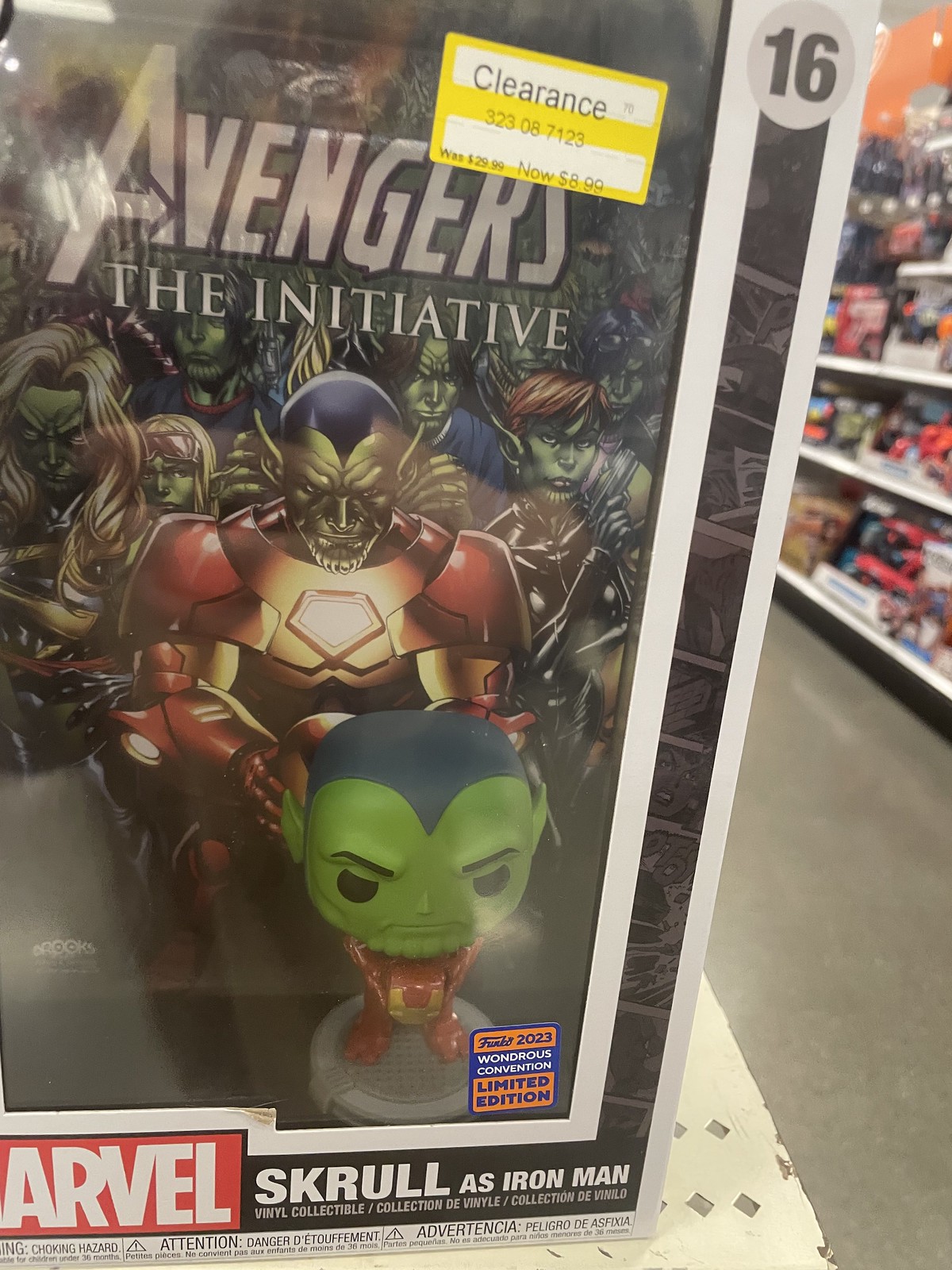The image is a detailed color photograph of a Funko Pop packaging displayed on a shelf in a store. The packaging prominently features the Marvel character, Skrull as Iron Man, from the Avengers: The Initiative series, with a number "16" marked along the right side and a Marvel logo at the bottom. The Funko Pop figure inside displays a green face with a top navy blue head and is attired in an Iron Man-inspired suit. A yellow clearance sticker on the front indicates that the price has been reduced from $29.99 to $8.99. Additional labels on the box include "Limited Edition" and "Wondrous Convention Limited Edition 2023." The background highlights various Avengers characters, including a robotic figure resembling Iron Man with red shoulder pads and a gold face, emphasizing the collectible nature of this item. Behind the main package, toy-laden shelves and a gray floor aisle are partially visible, situating the item clearly within a retail environment.